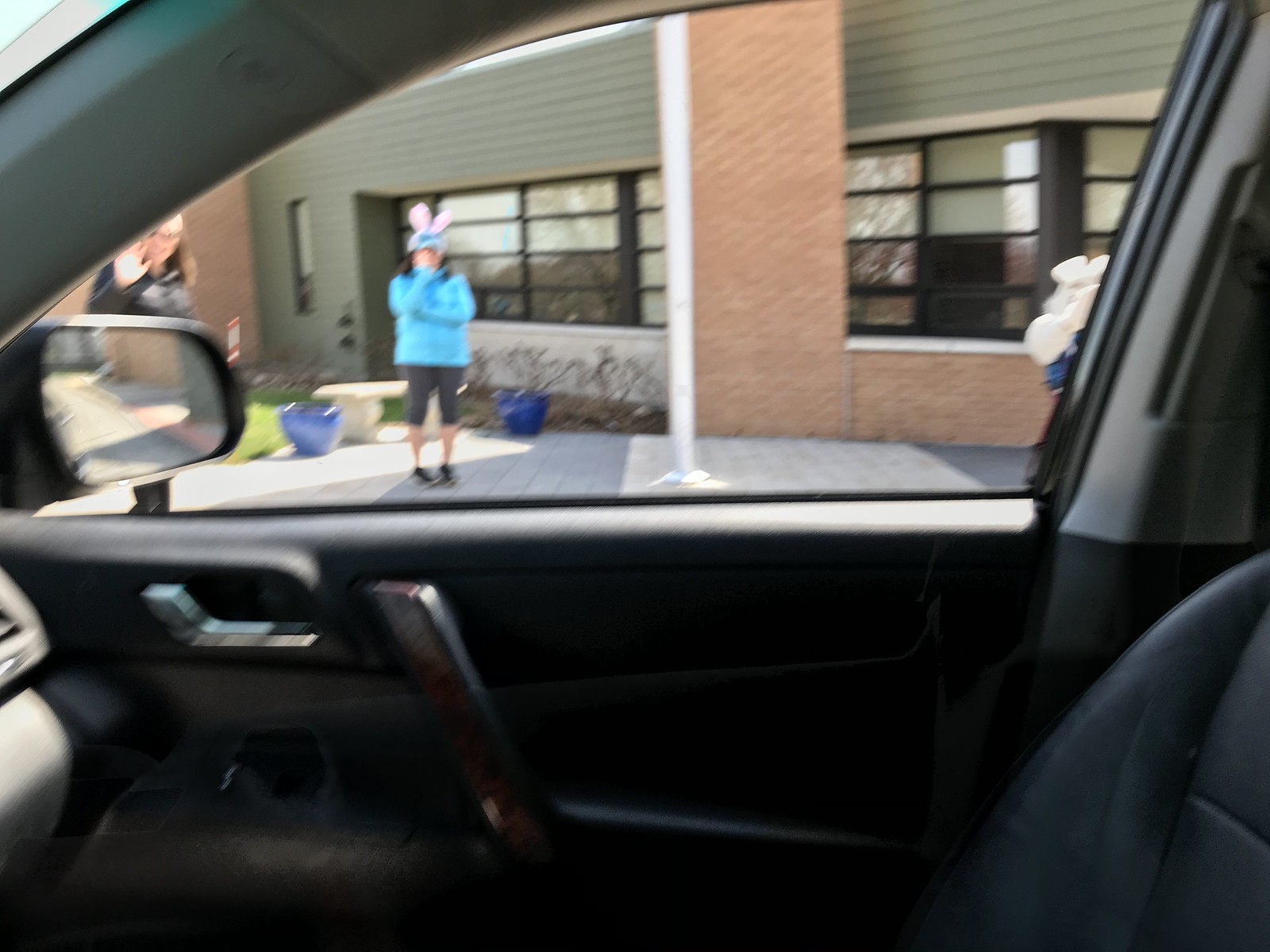In this image, the view is captured from the passenger side of a car with a rolled-down window showcasing the vehicle’s black interior. Outside the car, a girl stands on a walkway in front of a building that appears to be a school. She is dressed in a long-sleeved blue sweater and shorter black pants, complemented by black shoes. Close to her, two blue buckets suggest recent gardening work near some plants. The building behind her features a partial brick facade transitioning to light gray walls with numerous windows. Additionally, next to the car window, there are rolls of a white material, possibly paper or fabric. In the background, another girl wearing a black coat is seen walking and waving.